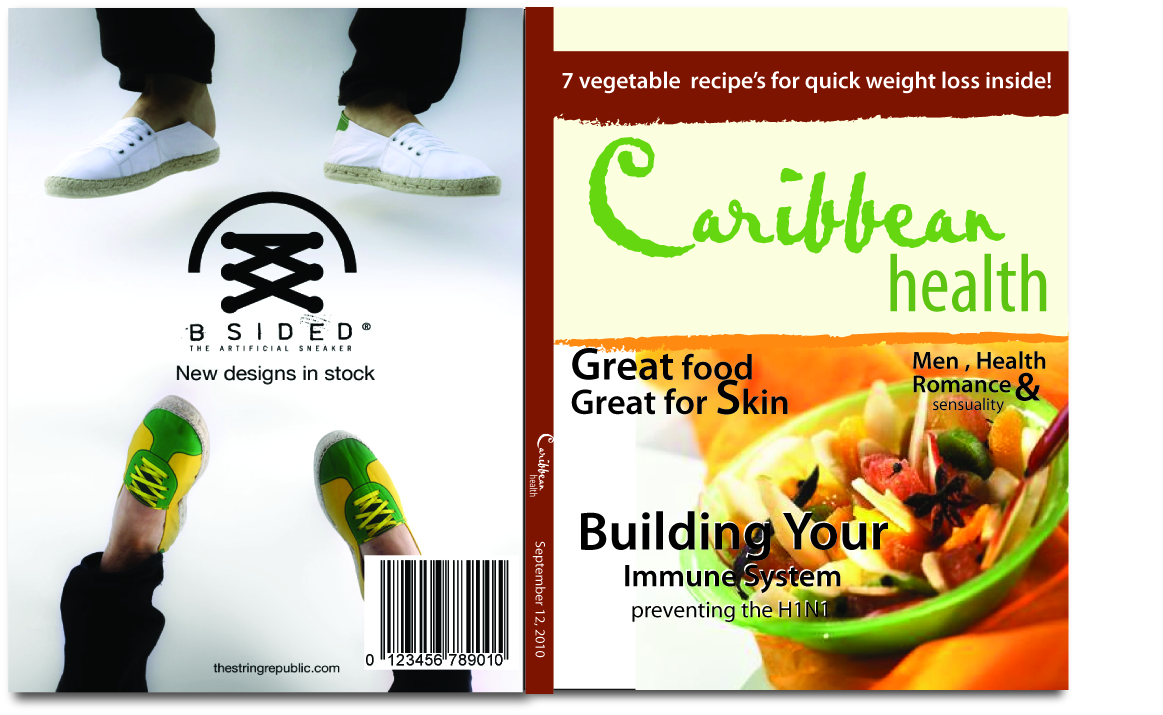This image features an open book or magazine showing both the front and back covers. The right side displays the front cover titled "Caribbean Health" with a green band across the top that reads "7 Vegetable Recipes for Quick Weight Loss Inside." The brown spine extends into this green band. Prominent text on the front cover includes "Great Food, Great for Skin" at the bottom and "Men, Health, Romance, and Sensuality" on the right. A green bowl filled with fruit and vegetables is featured prominently, atop which reads "Building Your Immune System, Preventing the H1N1."

The left side of the image, showing the back cover, features an advertisement for shoes with a photo depicting what seems to be a man's feet in white shoes and a pair of women's feet in green and yellow shoes below. The ad text reads "Be Sighted, New Designs in Stock." A barcode and the URL "StringRepublic.com" are located at the bottom right of the back cover. The layout is unusual as it appears the covers were removed from the book or magazine and laid flat for the photograph.